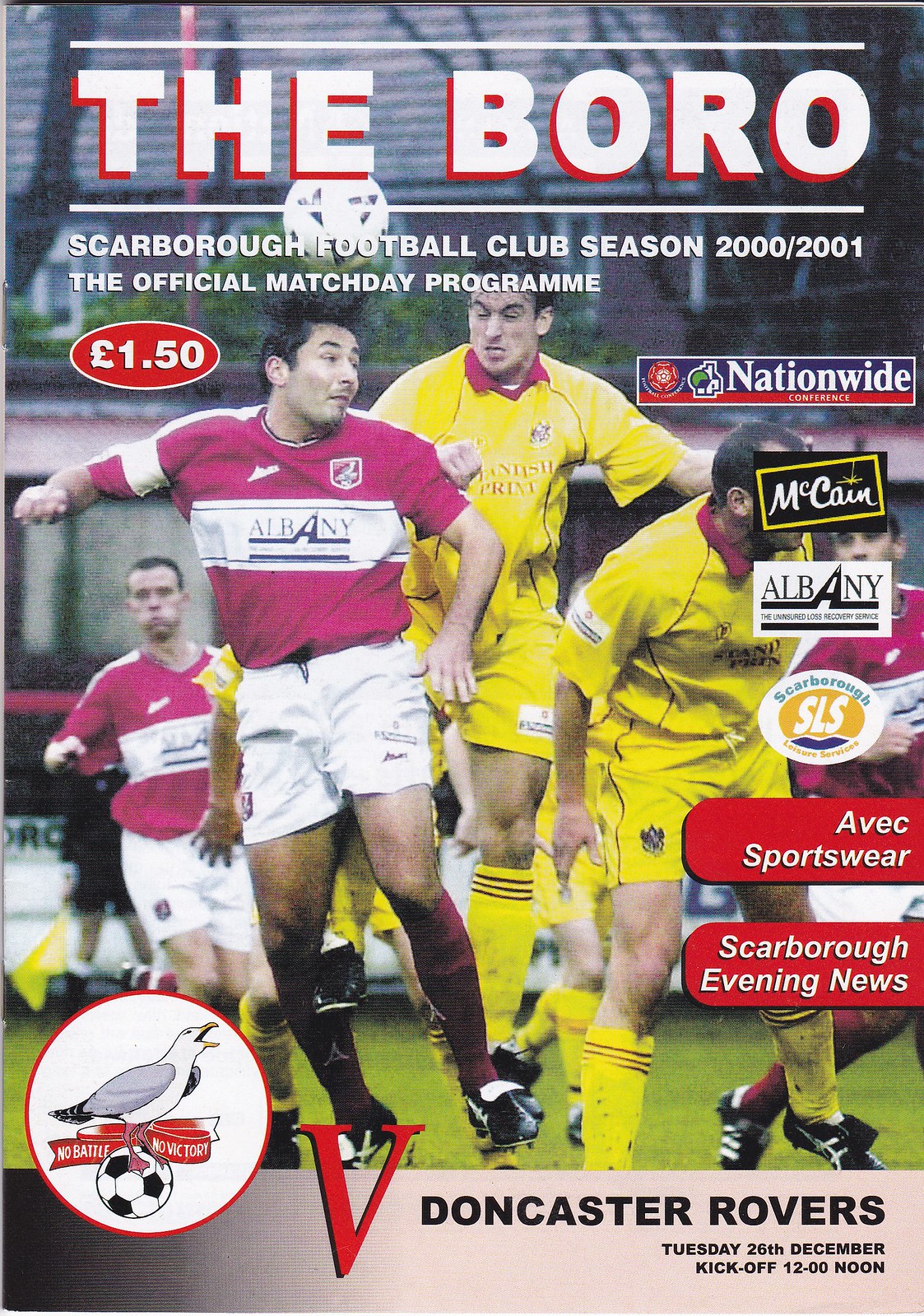The cover of the program for the Scarborough Football Club's season 2000/2001 match against Doncaster Rovers is vividly adorned with colorful and detailed imagery. Dominating the top is the title "THE BORO" in bold, white, all-caps text with a red-hued shadow, underlined by the smaller text, "Scarborough Football Club Season 2000/2001 The Official Match Day Program," also in white. An oblong text box indicates the price of the program as "£1.50."

The background features an action-packed, full-color photograph of a soccer match between two teams. On the left, a player from the Scarborough team, identifiable by his burgundy jersey with a white stripe and labeled "AIRMATE" across the front, is leaping to head the ball. He is paired with another player in a burgundy uniform on both the far left and right sides of the scene. Opposing them are players in yellow jerseys with red accents, also jumping to compete for the ball.

The right-hand side of the cover showcases several sponsorship logos, including those for Nationwide, McCain, Albany, Scarborough SLS, AVEC sportswear, and the Scarborough Evening News. A red, rounded, rectangular-shaped text box nearby emphasizes "No Battle, No Victory" with a bird standing atop a soccer ball.

The bottom banner of the cover provides essential match details, reading "V Doncaster Rovers, Tuesday 26 December, Kickoff 12 o'clock noon."